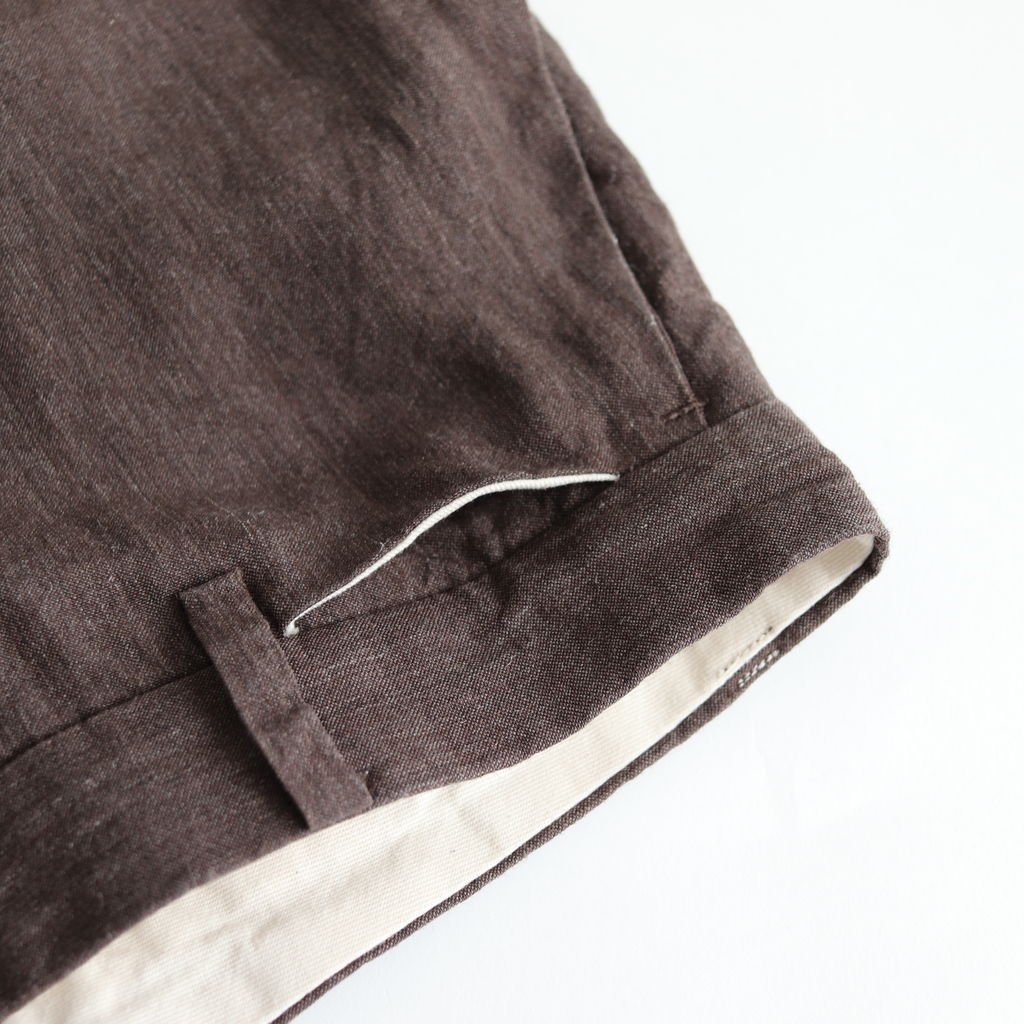This image features a close-up view of a pair of brown dress pants, likely intended for wearing with a suit. The photograph is highly zoomed in, focusing on the waistband area and part of a pocket, including detailed stitching. A single belt loop is visible in the bottom left corner of the image. The pants are draped on an off-white surface, and a light inner lining is faintly visible around the waist and pocket area. The object occupies the upper left, lower left, and the central sections of the frame, leaving much of the pants cut off by the edges of the image. The fabric appears to be a fine-knit material, and there are some small fuzzies present on the fabric, suggesting the pants may be gently used. This level of detail likely serves to highlight the texture and quality of the material, typical for a clothing item showcased on an online retail platform.